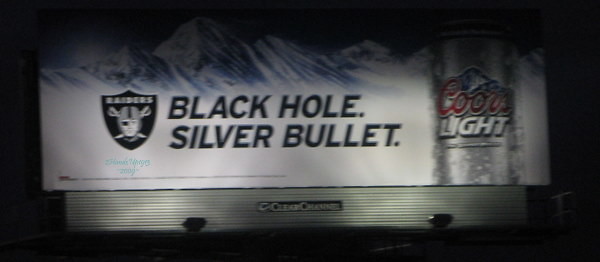In this low-quality, out-of-focus nighttime photograph, a Coors Light Beer billboard takes center stage. The billboard prominently features a can of Coors Light on its right side. In the middle of the billboard, the words "Black Hole, Silver Bullet" are boldly displayed. To the left, the iconic Oakland Raiders mascot is visible, depicted with its typical character—a face within a black, shield-like emblem. The background of the billboard showcases a classic blue and white icy mountain range, a common element in Coors Light advertising. Two physical lights point towards the picture taker, and an additional light shines up to illuminate the billboard. Surrounding the billboard is the pitch-black darkness of the night.